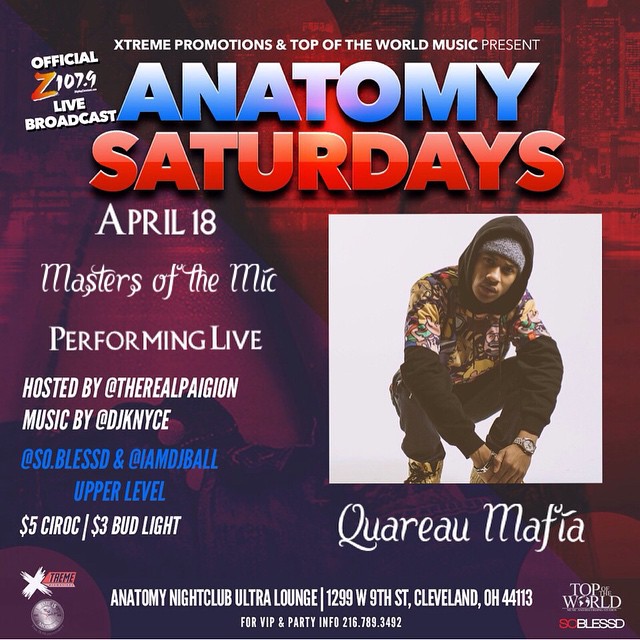This advertisement flyer promotes a live musical performance on Saturday, April 18th, titled "Masters of the Mic," to be held at Anatomy Nightclub Ultra Lounge, located at 1299 West 9th Street, Cleveland, Ohio, 44134. The event is hosted by The Real Paijun and features music by DJ Kyn(e) and DJ Nice. 

The flyer, backed by sponsors Z107.9 and promotional companies Xtreme Promotions and Top of the World Music, prominently displays "Anatomy Saturdays" with "Anatomy" in blue and "Saturdays" in red text. It also highlights a live broadcast by Z107.9.

A central image features a black artist named Quaray Mafia, dressed in a black hoodie under an anime-themed shirt, a gray beanie, dark pants, and brown boots. He is also seen wearing a silver wristwatch on his left hand and a silver bracelet on his right, set against an all-white background.

Additional details note a $5 upper-level entry fee, $3 Bud Light specials, and promotions by both Xtreme Promotions and Top of the World Music, whose logos appear at the bottom right of the flyer. VIP and party information can be accessed by calling 216-789-3492.